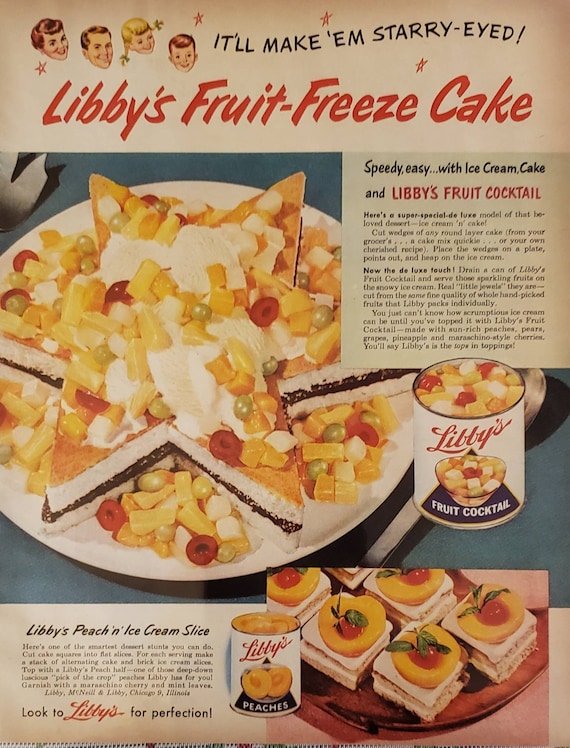This vintage advertisement from Libby's, likely dating from the 1950s or 60s, promotes their Fruit Freeze Cake. At the center, a six-pointed star-shaped cake takes the spotlight, adorned with a generous serving of classic fruit cocktail, including cherries, peaches, pears, and pineapples, all topped with whipped cream and possibly ice cream. The vibrant red letters at the top spell out "Libby's Fruit Freeze Cake," and whimsical 50s-style clipart of a family—comprising a wife, husband, pigtailed blonde girl, and short-haired boy—adds nostalgic charm with the tagline "It'll make them starry-eyed" surrounded by twinkling cartoon stars. The bottom of the advertisement features a variation of the dessert called "Libby's Peach and Ice Cream Sickle Slice," which appears as squares, along with a can of Libby's fruit cocktail used in the recipes. The entire page, with its slightly faded photo, exudes a retro appeal, evoking memories of mid-20th-century culinary delights.